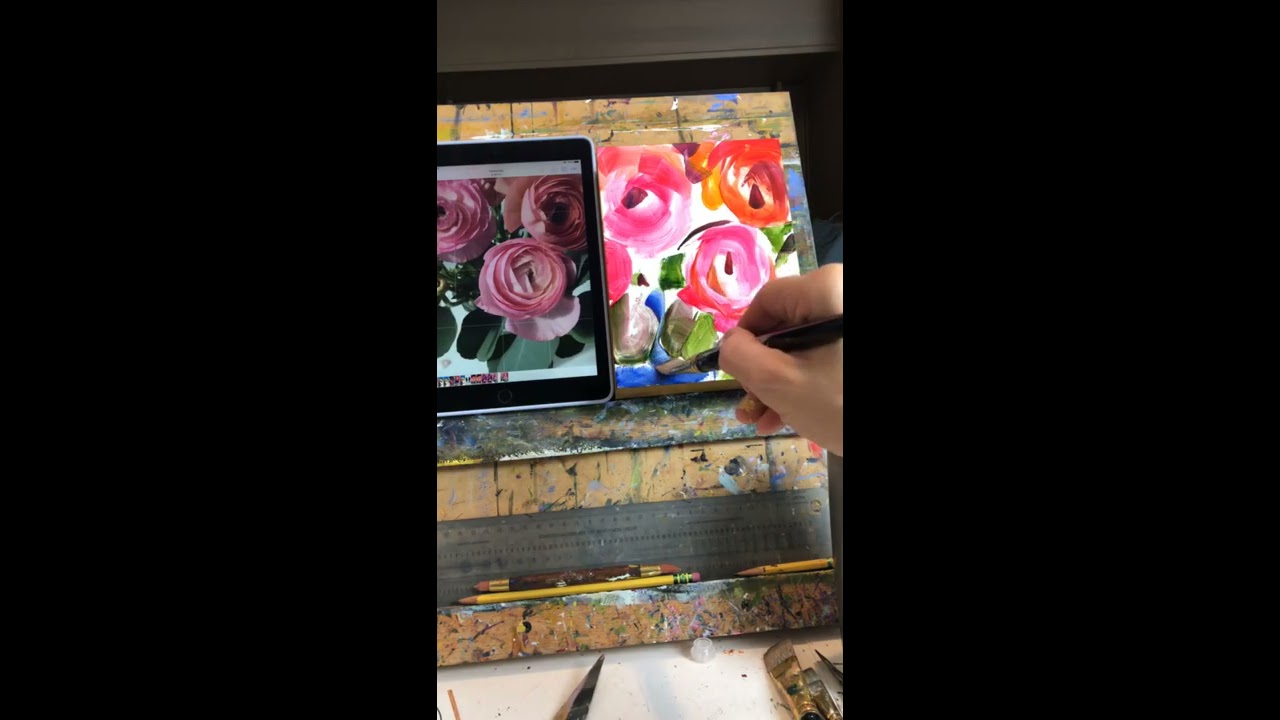In the horizontal-rectangular image, there are wide black borders on either side framing a narrow center photograph. The scene depicts an artist in the process of painting, with a focus on a piece on an easel. The easel appears to be makeshift, constructed from rough wood akin to a barn door. Propped up to the left side of the easel is a tablet displaying a reference photograph of three roses with surrounding foliage, which the artist is meticulously replicating. The artist's hand is poised with a paintbrush, actively painting a blue border across the bottom portion of the piece. Below the easel lie various tools, including paintbrushes of different sizes, chisels, a ruler, and a couple of pencils, indicating a well-used workspace. The painting already shows splatters of multiple colors, suggesting a vibrant, creative process. The entire setting hints at an indoor studio environment, though the exact location remains unspecified.